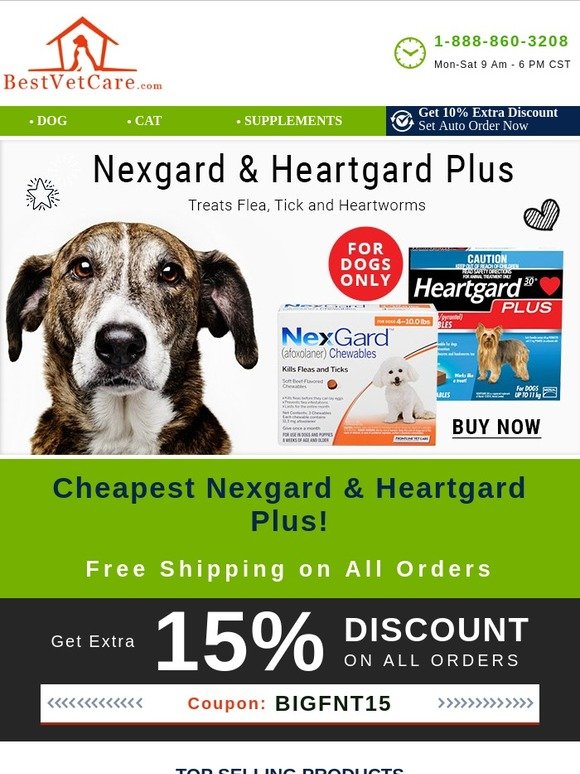Title: Best Pet Care - Premier Pet Health Solutions

Caption:
This screenshot features the homepage of BestPetCare.com, a veterinary care website. The top-left corner displays the site's name in bold red font, complemented by a doghouse-shaped logo with an adorable dog inside. Situated to the right are a green clock icon and a phone number, 1-888-860-3208, both matching in color. The operational hours, listed in green text, indicate the vet care services are available Monday to Saturday from 9 AM to 6 PM CST.

A prominent green navigation bar spans the width of the page, transitioning to dark blue on the right. The green section includes categories for "Dog" and "Cat," each marked by two dots, and "Supplements" with a single dot. The dark blue section features a checkmark logo icon and the enticing phrase "Get 10% extra discount" in white lettering.

Directly below, larger letters announce the availability of NextGuard and HeartGuard Plus, with smaller grey text detailing their use: "Treats Flea, Tick, and Heartworms." Decorative elements, including a star to the left and a heart to the right, add a touch of charm.

A central image showcases a friendly brown and white dog with expressive brown eyes and a white-tinged nose and neck, facing the camera. To its right, a red circle with white all-caps text reads "FOR DOGS ONLY." The image prominently highlights a NextGuard Chewables package and HeartGuard Plus box. The NextGuard package features a white poodle, while the HeartGuard Plus box, colored black, red, and blue, depicts a brown Yorkie with "Buy Now" written in black below.

A green bar beneath this section states in blue text, "Cheapest NextGuard and HeartGuard Plus," and promises "Free Shipping on All Orders" in white. Further down, a black banner promotes an additional discount: "Get Extra 15% Discount on All Orders," with the "15%" prominently enlarged. A coupon code "BigFNT15" is highlighted in a red coupon bar with arrows pointing left and right, emphasizing the offer.

This detailed homepage snapshot underscores Best Pet Care's commitment to providing exceptional pet health solutions and promotions for pet owners.